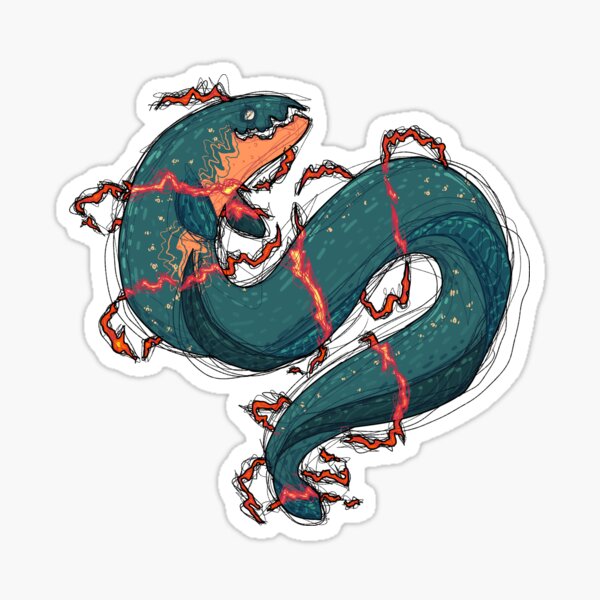The image depicts a vividly illustrated sea creature resembling an eel, coiled in an S-shape. The creature is characterized by a deep aquamarine or dark teal hue, with a notable feature being its underbelly, colored a contrasting flame-like orange. Red, zig-zaggy lines spiral around its body, suggestive of electricity, extending from its head to the tip of its tail. The eel's mouth is slightly open, revealing sharp white teeth, and it has small fins near the upper part of its body. The artwork appears to be a detailed, cartoon-style drawing and is likely a sticker, as indicated by the matching outline around the eel against a white background, suggesting it can be peeled and affixed to surfaces.